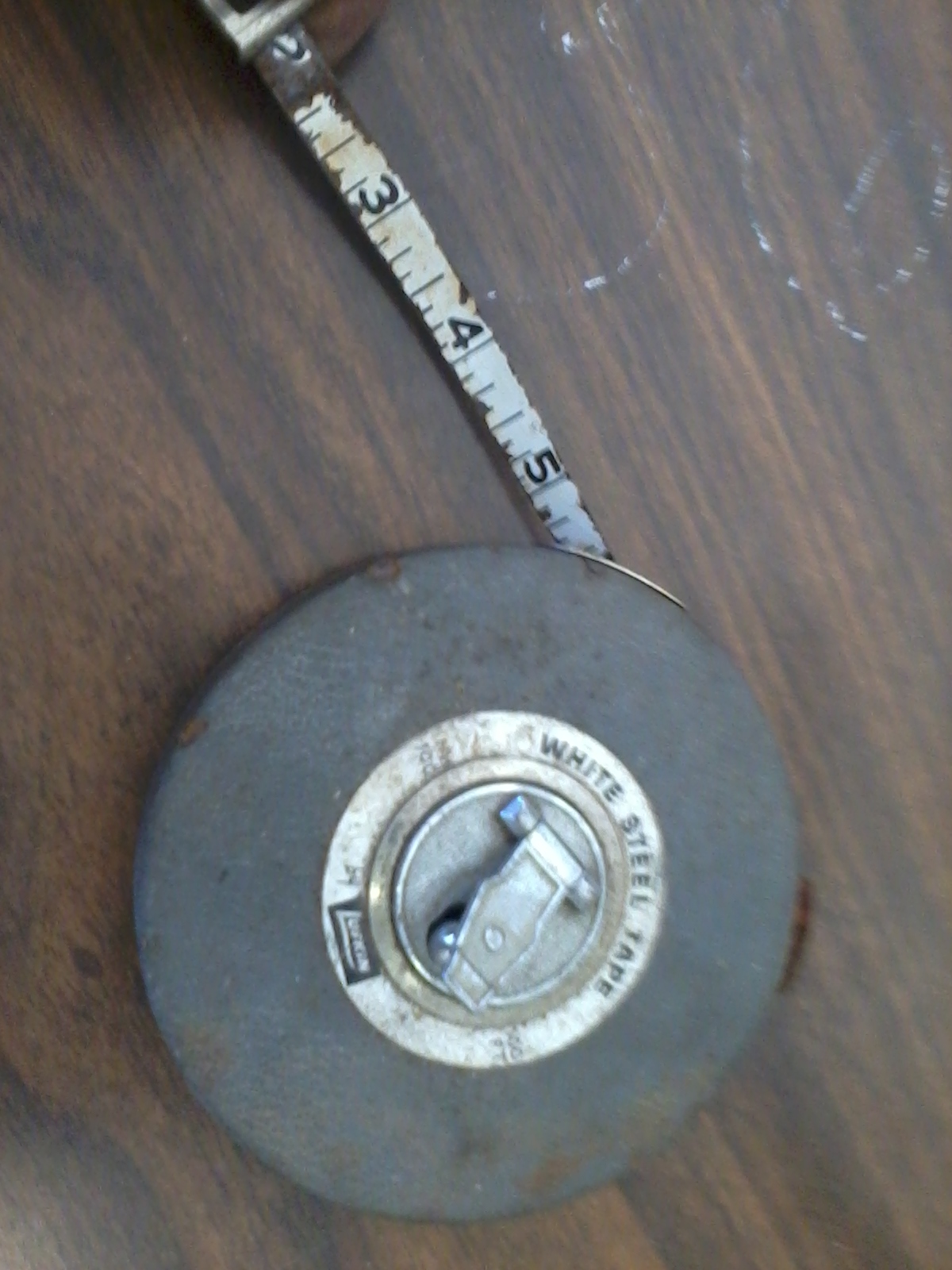This close-up photograph features a large, worn tape measure, typically used in construction, lying on a brown, possibly laminate, wooden table. The table's surface presents slight white marks or possible paint splatters on the top right-hand side. The tape measure's tape is white, rusted, and we can clearly see the numbers 3, 4, and 5 along with the inch, quarter inch, half inch, and eighth inch markings. The device itself is encased in a black metal drum, accented with a white circle displaying the label "White Steel Tape" in black letters and a logo beneath that seems to say "Luffman" in white. A brass metal handle, which is folded into the drum, can be pulled out and twisted to wind or unwind the tape. This sophisticated yet aged tool, with light grey and silver accents, reflects its well-used nature and essential role in precise measurements.